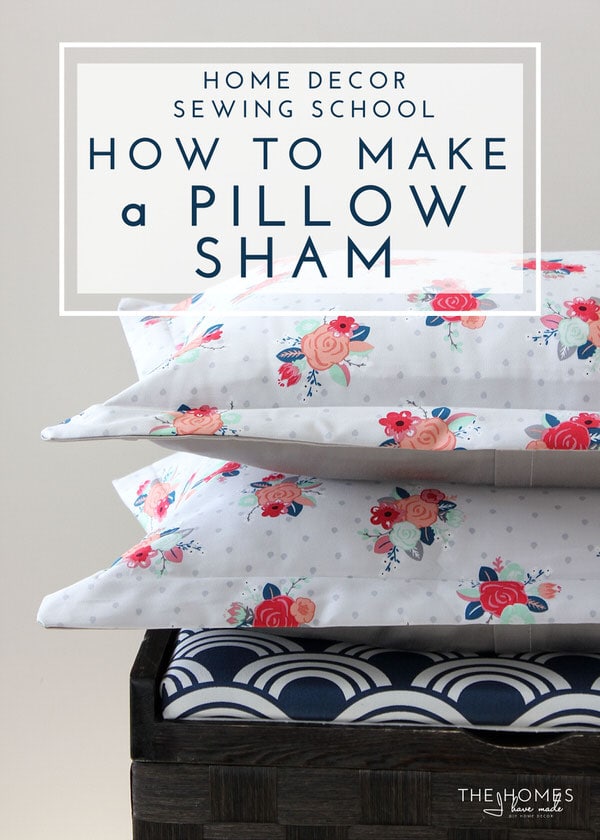The image depicts an advertisement poster for a class titled "Home Decor Sewing School: How to Make a Pillow Sham." The central feature of the poster is a beige rectangle with a slightly transparent overlay, showcasing the course title in dark blue, all-capital letters. Below the title, two pillows are neatly stacked atop a scallop-patterned seating area of a wooden bench, partially visible at the bottom right of the image. Each pillow features a floral design with an array of pink and dark pink flowers, coupled with blue and teal leaves on a white background with gray polka dots. Another cushion with a navy and white abstract pattern lies underneath the pillows. In the bottom right corner, the text "The Homes I Have Made" is inscribed, possibly accompanied by an indistinct signature that might read "J Handmade."